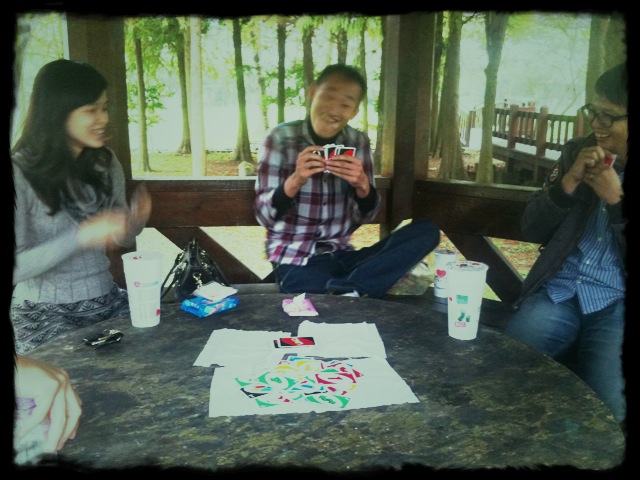The photograph, rectangular in shape with longer top and bottom sides, captures a moment of leisure with three individuals engaged in a game of UNO around a brown and black round stone table. A black border on all four edges gives the image a burnt appearance, while a yellowed filter adds an aged, nostalgic feel. The overall image is slightly out of focus, contributing to its vintage aesthetic. 

In the center of the image, a person sits with their leg propped on their right knee, dressed in dark blue denim jeans and a distinctive purple, white, and black plaid shirt over a long-sleeved black shirt. Their sleeves are slightly pushed down to the forearm, and they hold several UNO cards in both hands. 

To the top right, another individual wearing blue denim jeans is seen in a white and blue striped button-up shirt layered under a gray jacket, accessorized with glasses that hint at a thoughtful demeanor. 

At the top left corner, the third player is comfortably clad in a gray and white skirt paired with a long-sleeved gray top. 

Set outdoors, likely in a park, the relaxed and joyful atmosphere is subtly captured despite the slight blur, portraying a timeless scene of camaraderie and fun.